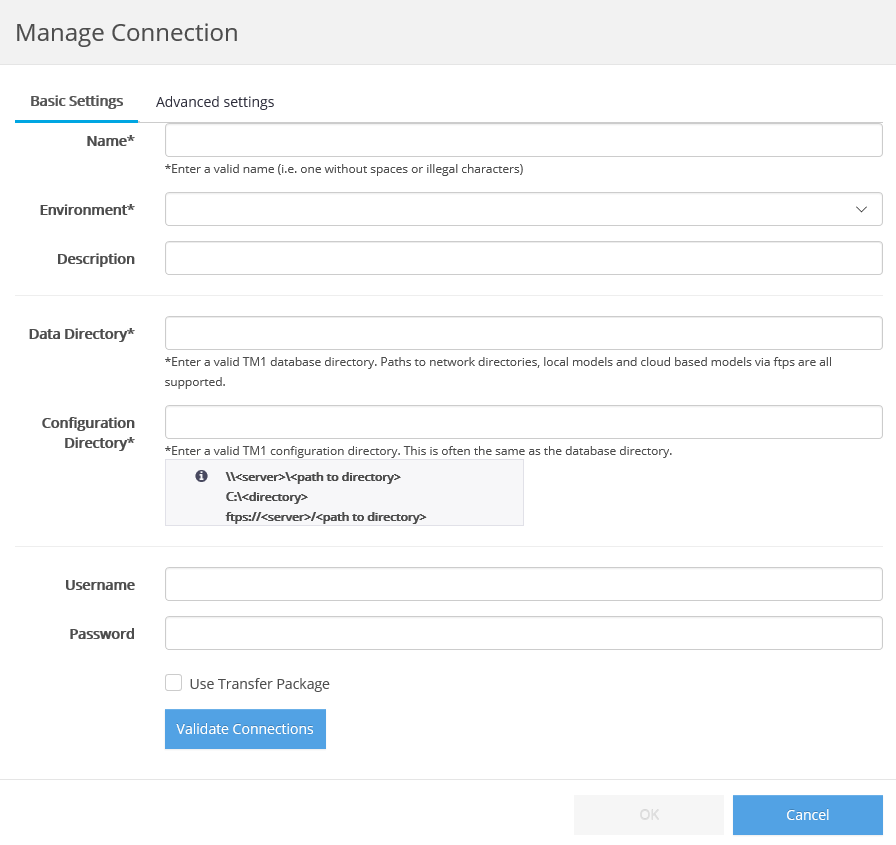The image displays a user interface titled "Manage Connection," highlighted in black text against a gray background. Below the title, there are two tabs: "Basic Settings," which is underlined in blue and displayed in a darker gray to show it's selected, and "Advanced Settings."

Under the "Basic Settings" tab, the following fields and instructions are visible:

1. **Name**: Accompanied by an asterisk indicating a required field, with a tooltip reading "enter a valid name, i.e. one without spaces or illegal characters." The input field is white and blank.
2. **Environment**: An empty input field.
3. **Description**: Another empty input field.
4. **Data Directory**: A blank input box with the instruction "enter a valid TM1 database directory. Paths to network directories, local models, and cloud-based models via FTPS are all supported."
5. **Configuration Directory**: Accompanied by a message explaining that it should contain a valid TM1 configuration directory, often the same as the database directory. Below this, there is a grey box displaying an example configuration path or code snippet.

Further down, there are fields for **Username** and **Password**, both of which are blank.

An option to **Use Transfer Package** is present, followed by a blue "Validate Connections" button.

At the bottom-right of the interface are two buttons: "OK" in gray and "Cancel" in blue.